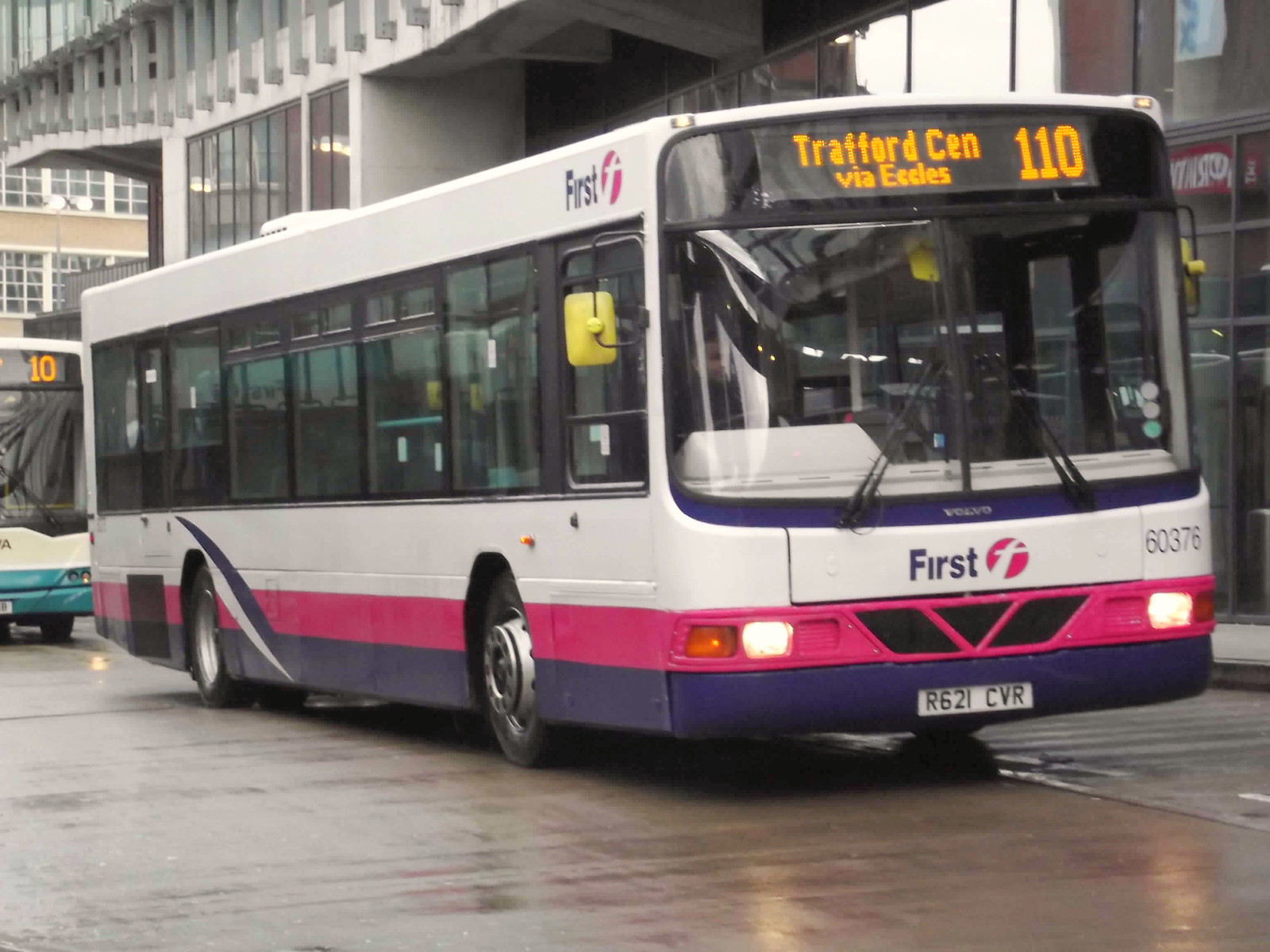A white city bus from the transportation company "First" is parked on a wet asphalt street, suggesting recent rain. The bus prominently displays its destination on a lit-up sign that reads "Trafford Center via Eccles 110." The front windshield is split down the middle by a black line, with wipers angled inward. Below the windshield, a pink bumper and headlights are visible. A red circular logo with a white "F" is positioned beside the large text "First," and the bus route number "60376" is found near the edge. A white license plate reads "R621 CVR."

The bus features tinted windows with black frames, a pink stripe running the length of the bus near the bottom, and a purple stripe underneath. A yellow rear section with a mirrored finish can be seen on the side. Ahead of this bus is a glass-fronted building, hinting at a commercial or transport hub. Another bus with a blue bumper and labelled "10" is visible in the background.